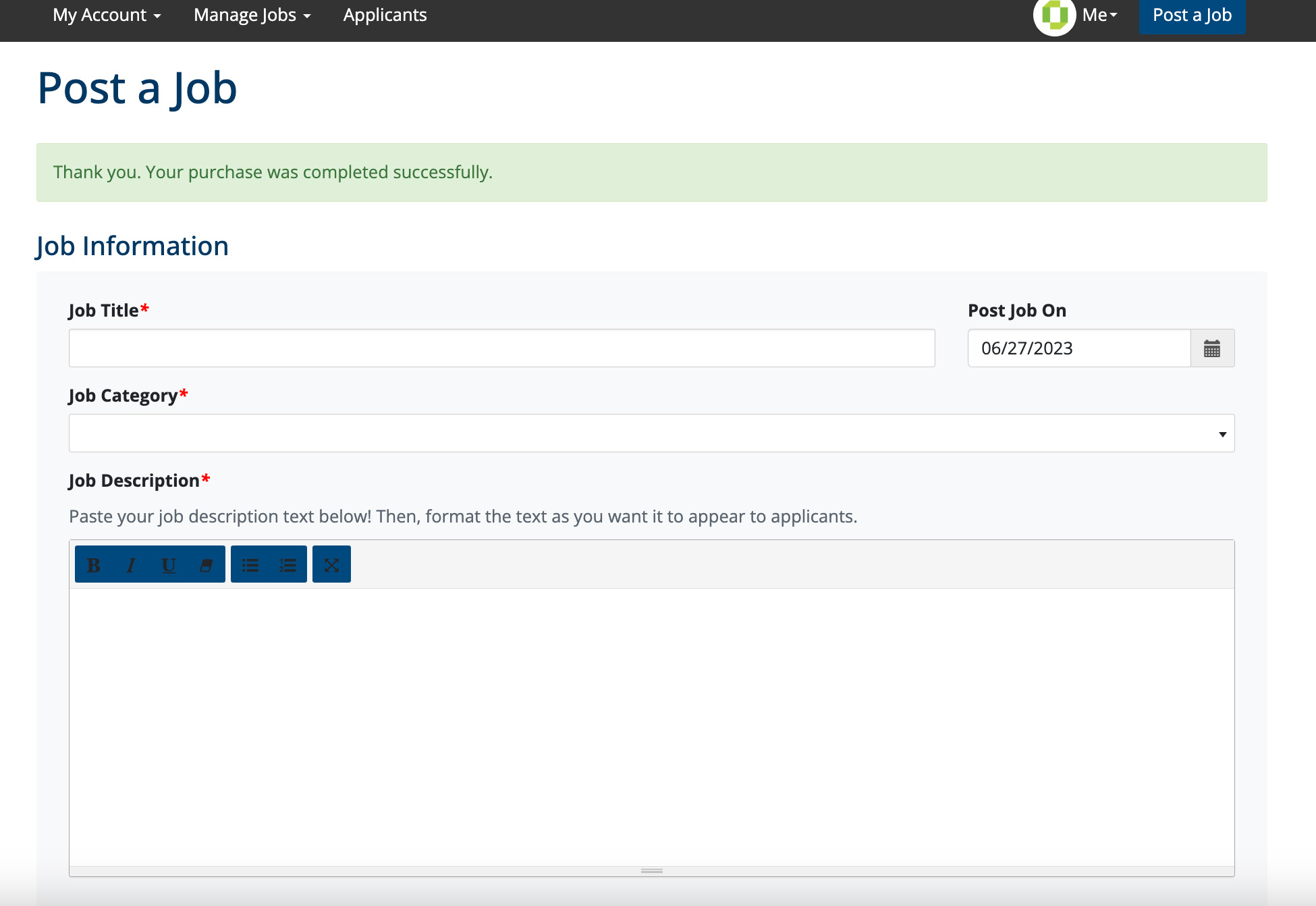A detailed screenshot of a job posting dashboard features an organized layout for users to create and manage job listings efficiently. The top of the page sports a black navigation bar with menu options including "My Account," "Managed Jobs," and "Applicants," alongside a prominent blue "Post a Job" button. Below, highlighted in blue, is a banner with the text "Post a Job," followed by a green confirmation stripe reading "Thank you, your purchase was completed successfully."

The main section presents a clear, structured form set against a light gray background with white text boxes. This form is titled "Job Information" and prompts users to fill in fields such as Job Title, Date Posted, Job Category, and Job Description. Beneath the Job Description field, instructions request users to paste their job description text and format it to appear as desired by applicants. The entire interface is clean and user-friendly, aiming to simplify the job posting process. The screenshot is noted to have been taken on June 27, 2023.